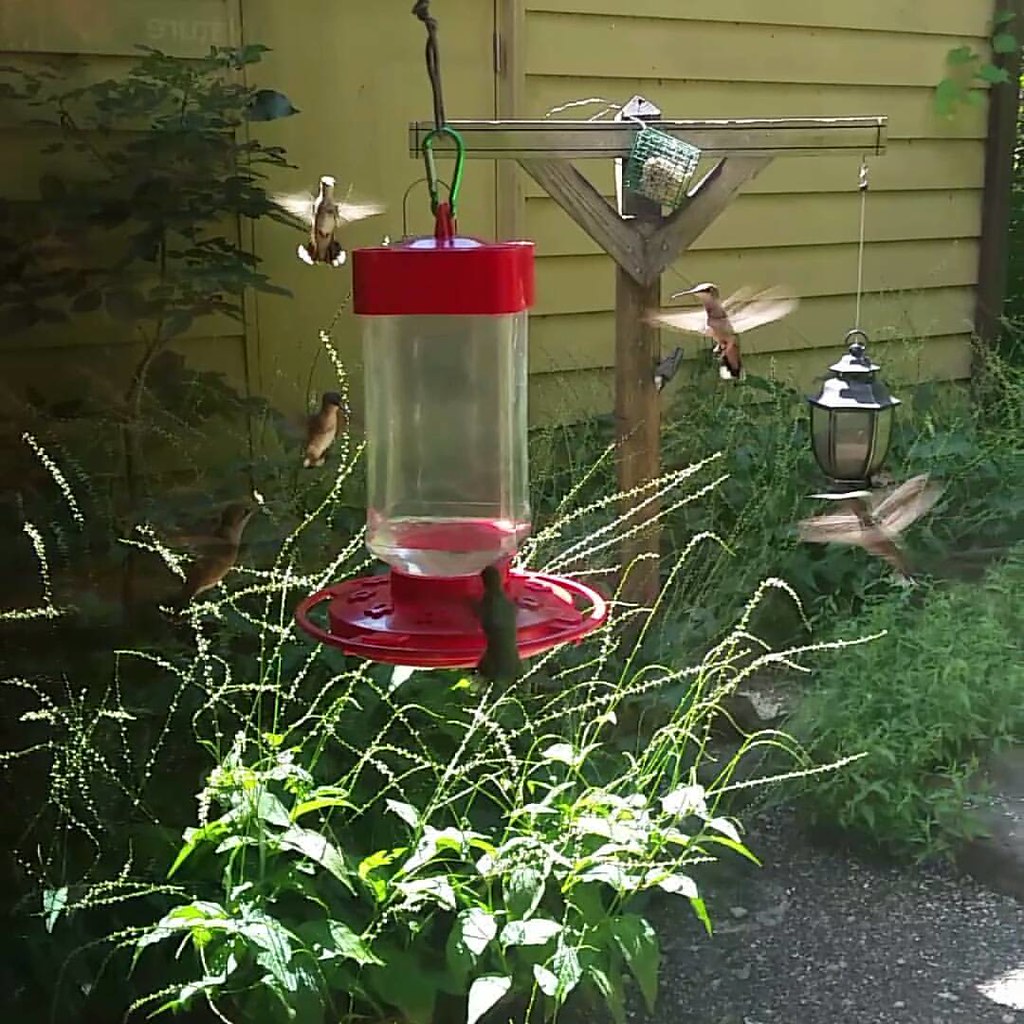The image features a vibrant scene centered around a hummingbird feeder hanging from a wooden post. The feeder has a vivid red top and bottom with a transparent plastic canister in between, showing some liquid at the base. Surrounding the feeder are several hummingbirds, some in swift flight with wings a blur, and others perched either on the feeder itself or nearby branches. The background reveals a garden lush with greenery, punctuated by a gravel path and a yellow shed. To the side of the wooden post, there is another bird feeder resembling a lantern, adding more charm to the picturesque setting. The scene is bathed in sunlight, capturing the lively atmosphere of the garden.